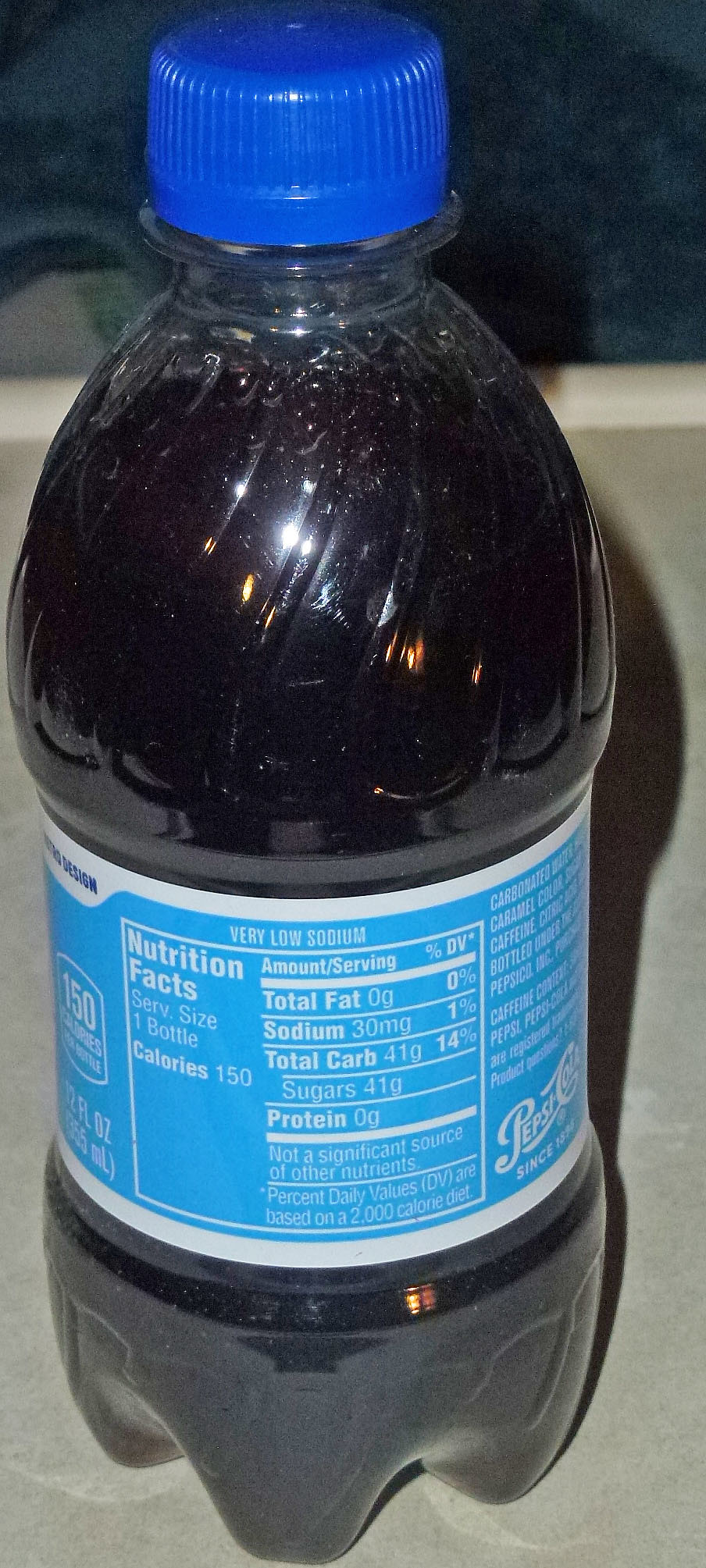This indoor photograph showcases an unopened, miniature 12-ounce bottle of soda. The bottle is capped with a cobalt blue lid, and it contains a very dark liquid that appears almost black in the image. The soda bottle features a vibrant medium blue label, accented with white lines along the borders. Prominently displayed on the label are the nutrition facts, which indicate the soda has 150 calories. To the right of these nutritional details, there is a Pepsi-Cola logo, accompanied by the text "Since 1895," though the exact year is somewhat difficult to decipher. Above the logo, a list of ingredients is visible. The bottle is situated on a gray-colored countertop, completing the setting for this detailed visual composition.